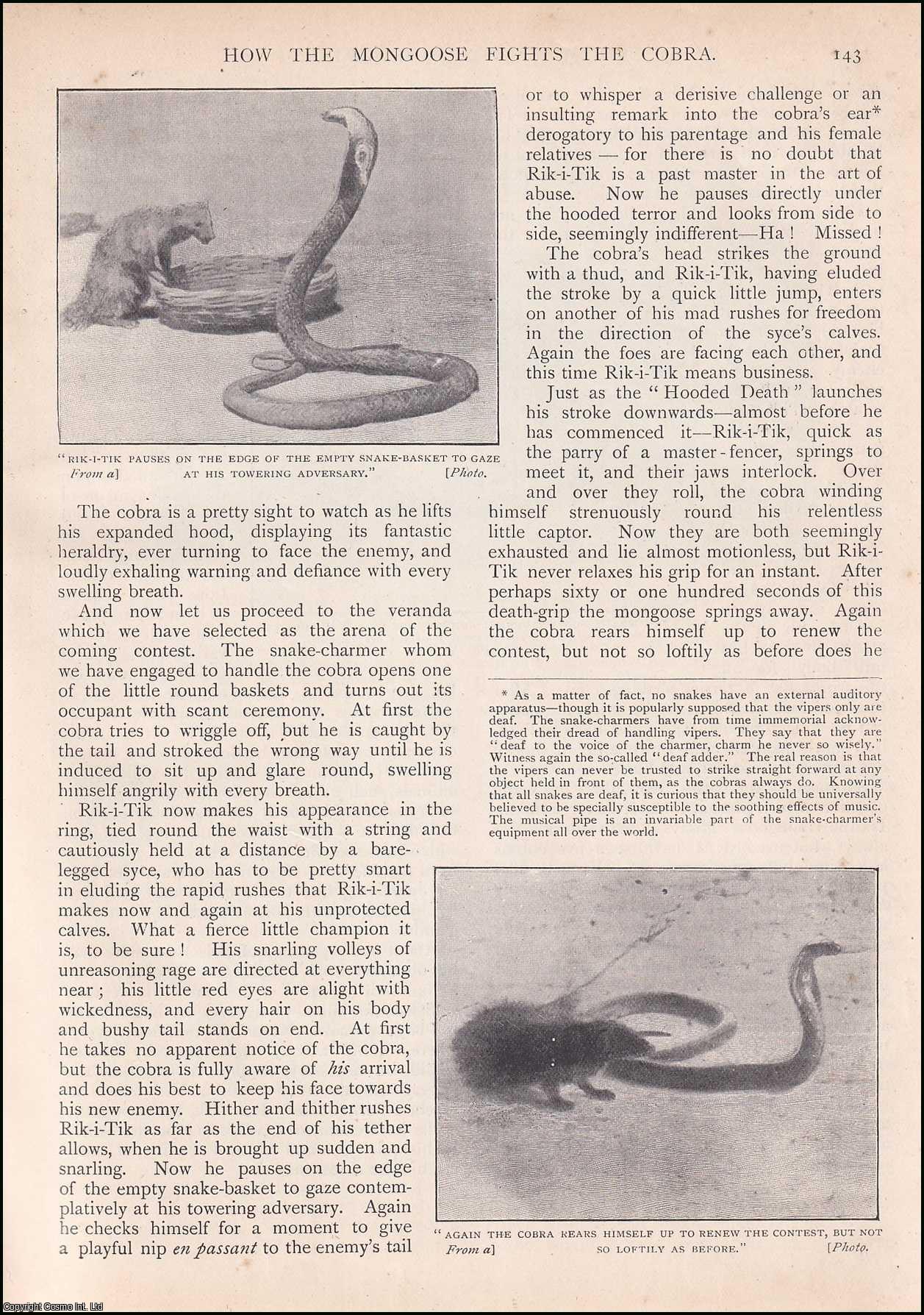This is a detailed black-and-white page numbered 143 from a book, featuring an article titled "How the Mongoose Fights the Cobra." At the top of the page, there's an image showcasing a dramatic standoff between a mongoose and a cobra. The mongoose is up on its hind legs with its paws on the edge of a straw basket, staring intently at the cobra, which has its hood expanded in a defensive posture. Under this top photo, the caption reads, "Rikki-Tikki pauses on the edge of the empty snake basket to gaze at his towering adversary." The page is adorned with large columns of text elaborating on the combat techniques between these two animals. Towards the bottom right of the page, there is another photo depicting the mongoose and cobra in mid-battle, with the caption, "Again, the cobra rears himself up to renew the contest, but not so loftily as before." The overall look of the page resembles a newspaper article, with its black-and-white print and yellowed appearance, contributing to its vintage feel.